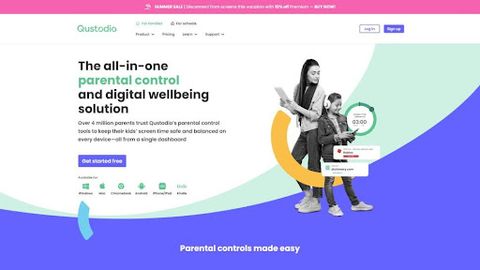The image features a promotional graphic for Qustodio, a parental control and digital well-being solution. Despite its poor resolution, the central message in bold, prominent text highlights that Qustodio is "the all-in-one parental control and digital well-being solution." It is accompanied by a reassuring statement that "Over 4 million parents trust Qustodio's parental control tools to keep their kids' screen time safe and balanced on every device from a single dashboard." 

The image includes a monochromatic photograph showcasing a woman and her child, both absorbed in their devices—a tablet for the mother and a phone for the child. The mother is shown glancing over her child's shoulder, symbolizing parental supervision. Stylized swoops of green and periwinkle blue adorn the background, with a striking pink strip across the top. Text in various colors including white, black, gray, yellow, green, and periwinkle navigate the viewer's attention through the visual design. 

The tagline "Parental controls made easy" is prominently featured, reinforcing the user-friendly nature of Qustodio's offerings. The image effectively conveys the brand's commitment to providing an accessible and comprehensive solution for managing children's digital activities.